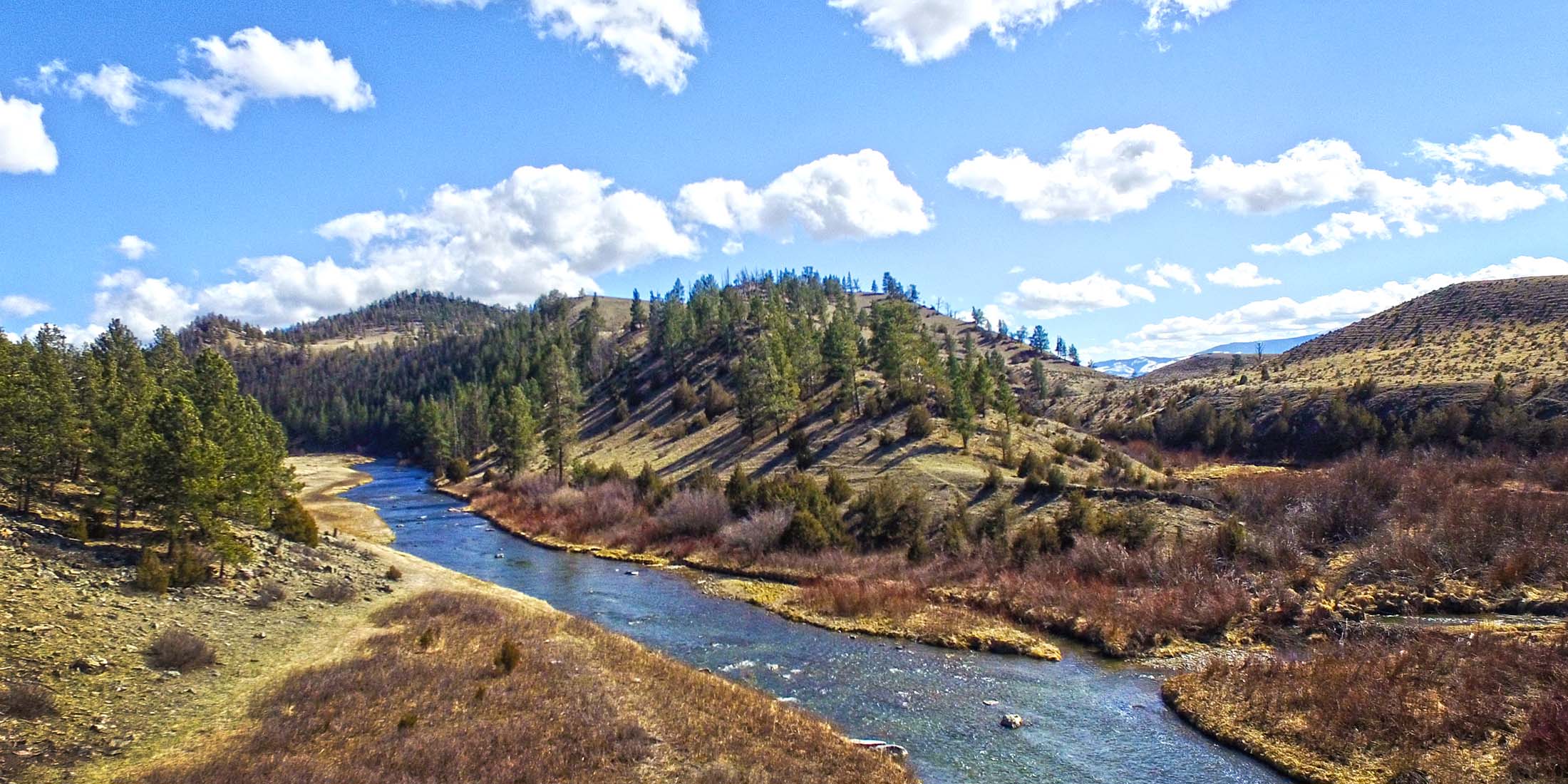The image captures a striking natural landscape, possibly reminiscent of the rugged terrains found in states like Colorado or Utah. It features a slightly rapid-moving blue river dotted with rocks, cutting through a varied terrain. The middle ground showcases a mixture of scraggy, dry brush and tufts of tall red and purple grass, blending with shorter shrubs. The river is bordered on one side by a barren hill scattered with smaller stumps and on the other side by lush green trees, including tall conifers. Farther back, small hills transition into a dense forest of mixed purple and green-leaved trees, indicating the changes of seasons, perhaps fall or spring. In the distance, a series of hills gradually give way to towering mountain ranges. The sky above is a clear blue, adorned with white fluffy clouds, enhancing the overall beauty and serenity of this remote, untouched landscape. There are no visible animals or people, emphasizing the pristine and isolated nature of the scene.